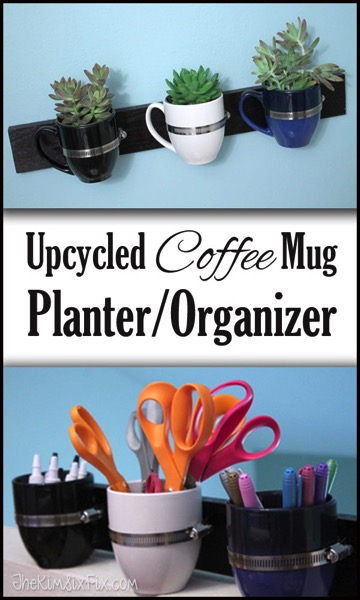The image is an advertising poster showcasing creative ways to upcycle coffee mugs into practical organizers and planters. Dominating the center is a white rectangle with black text reading "Upcycled Coffee Mug Planter/Organizer" in various fonts. Above the text, set against a pale blue background, are three coffee mugs—a black, a white, and a blue one—mounted on a wooden plank with metal bands. Each mug hosts a small succulent, blending utility with aesthetic appeal. Below the text, another photo displays a similar setup, but here, the three mugs are used to hold various stationery items such as pens, markers, and scissors. The mugs are again secured with metal bands, making them versatile holders mounted on the wooden board. The overall theme of the poster is sustainability and creativity, transforming everyday coffee mugs into functional and decorative home items.